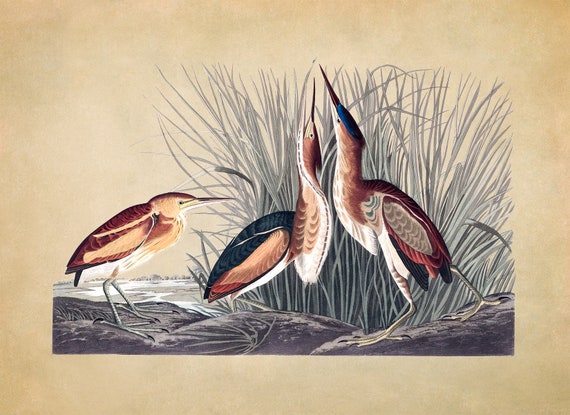This detailed illustration, likely a color plate from a book, depicts four birds resembling cranes, each meticulously detailed with pastel colors. The birds exhibit a diverse palette of feathers, including shades of brown, black, blue, white, and tan, as well as a striking magenta on one bird's wings. The bird on the far right stands apart with its bright red wings and blue head. Three birds in the center of the image have their beaks pointed skyward, poised in front of a tall patch of soft, grassy reeds in various hues of gray-green. To the left, another bird stands near a lake with rocks in the distance. The ground is dark, craggy, and adorned with small marks, adding to the image's intricate detail. The background features a light brownish and orange-yellow paper, lending a warm vintage feel to this richly colored and highly detailed depiction.